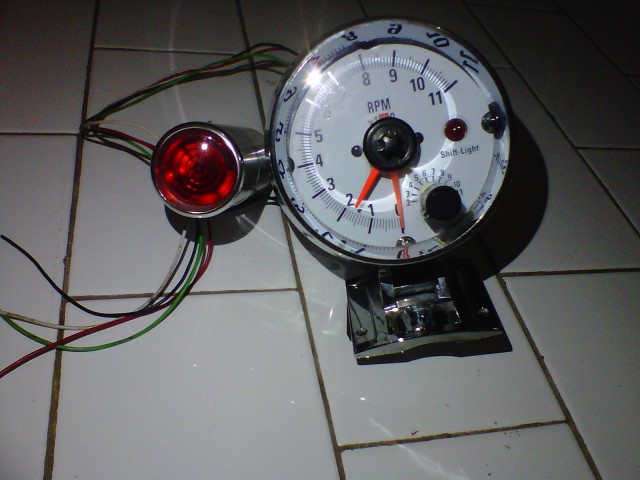The photograph showcases a mysterious circular device resting on a white tile floor with dark gray grouting. At first glance, it appears to be a clock, but upon closer inspection, it reveals itself to be something more complex. The face of the device is white and marked with numbers ranging from 0 to 11, accompanied by smaller gradation lines. The red hands, one longer and one shorter, suggest precision measurement, likely indicating RPM (revolutions per minute).

The device is labeled with various inscriptions, one of which suggests it has a red indicator light. Additionally, there's a small black knob featuring exceedingly small numbers, from 2 through 10, though the 1 is obscured. The central section from which the hands emerge is black, providing a stark contrast against the white face.

The top of the device appears to be covered in glass, reflecting ambient light. Emerging from the device are several wires—black, green, and red—that hint at an electrical component. A small, silver-toned piece with a prominent red light protrudes from the left side of the object, adding another layer of complexity to its function.